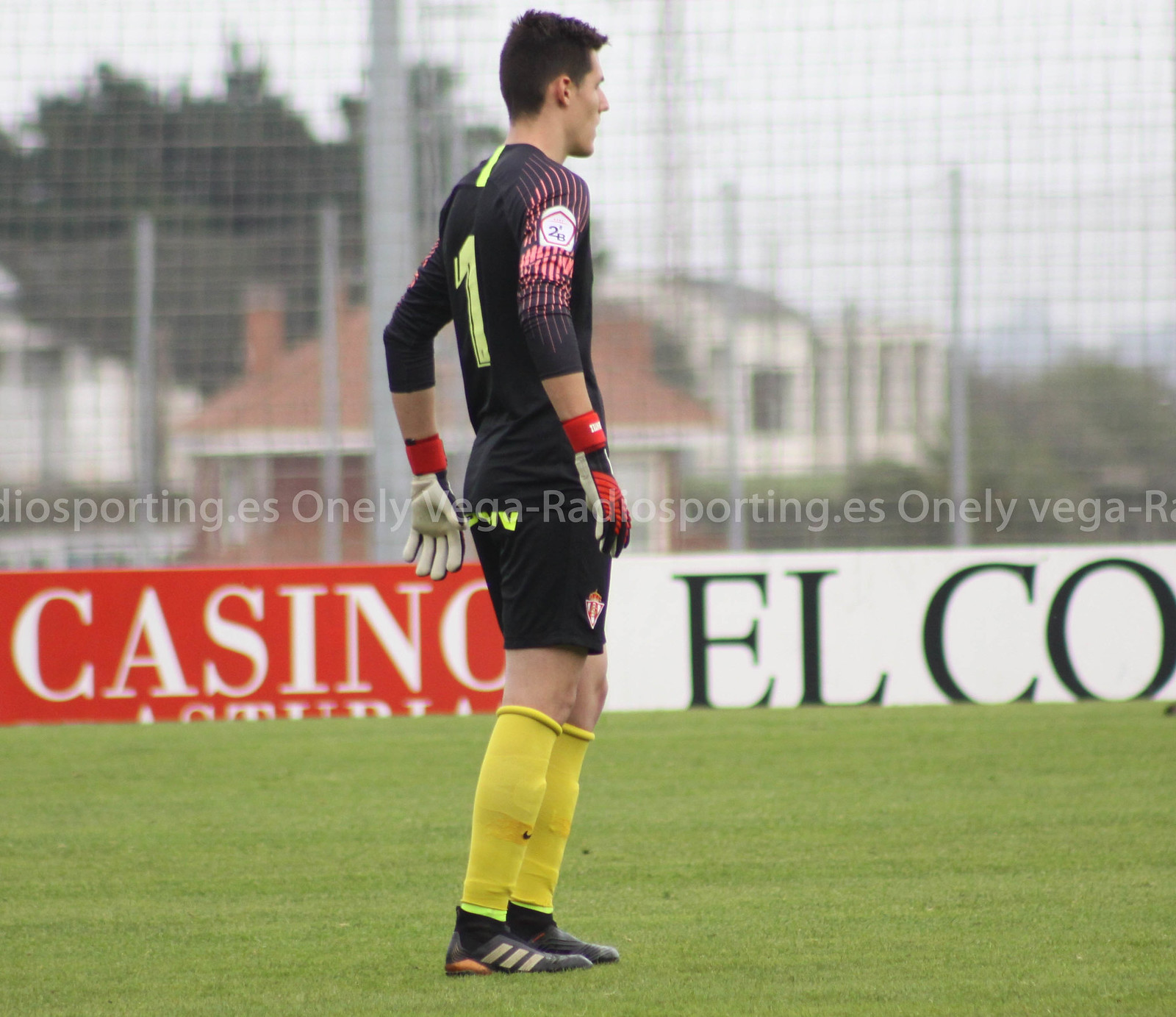The image depicts a soccer goalie on a vibrant green grass field, intently looking to the right as if anticipating the ball. The player has short brown hair and wears a black long-sleeved jersey with green number '1' on the back, complemented by black shorts. His gear includes yellow shin guards over green socks, and distinctive Adidas cleats featuring orange and gold stripes. The goalie is also equipped with white, red, and black gloves. In the background, a barrier adorned with advertisements—some clearly displaying "casino" and "Elko"—encloses the field. Beyond the barrier, a few brick buildings and trees are visible under a daytime sky.